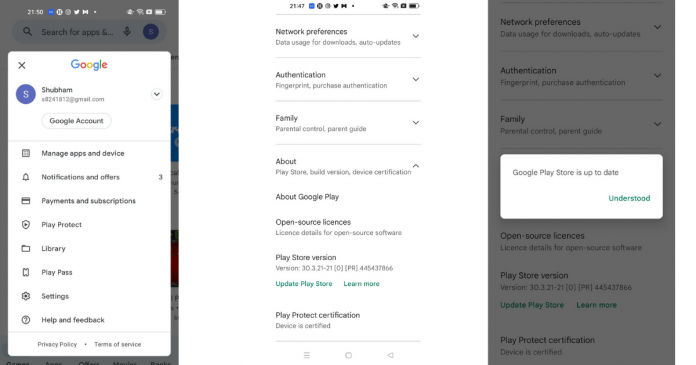The image consists of three different screenshots, each showcasing various settings pages within the Google Play Store application. 

On the left screenshot, the page displays the "Manage Apps & Device" section with a prominent white overlay that prompts the user for their email address at the top. It further lists several subsections including "Notifications & Offers," "Payments & Subscriptions," "Play Protect," "Library," "Play Pass," "Settings," and "Help & Feedback."

The central screenshot shows another segment of the Google Play Store settings. The top of this screen features categories such as "Network Preferences," "Authentication," "Family," "About," "About Google Play," "Open Source Licenses," and "Play Store Version." At the bottom, highlighted in green, are options to "Update Play Store" and "Learn More."

The rightmost screenshot includes a central white pop-up window informing the user that their Google Play Store is up to date, encapsulated in the simple message, "Google Play Store is up to date."